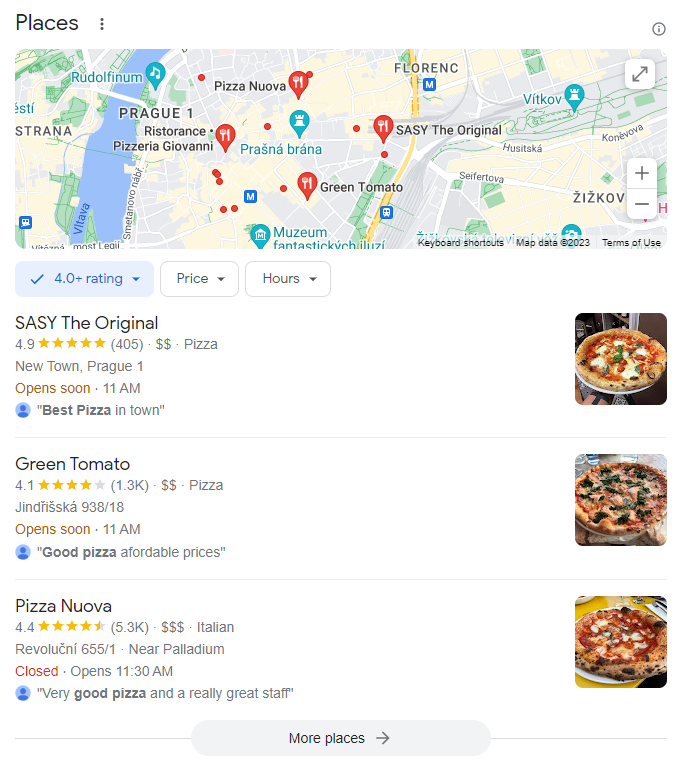This screenshot from Google Maps displays a map of Prague, highlighting various dining locations. Notable places marked on the map include Rudolfinum, Ristorante Pizzeria Giovanni, Pizza Nuova, Green Tomato, and SASY The Original.

Beneath the map, the details for each location are provided:
- **SASY The Original**: Rated 4.9 stars from 405 reviews, it offers pizza in New Town, Prague 1, with a price indication of two dollar signs ($$). It's described by reviewers as the "best pizza in town." The listing includes a photo of a Margherita pizza and notes that the restaurant opens soon at 11 a.m.
- **Green Tomato**: This spot has a 4.1-star rating from 1.3 thousand reviews, also priced at two dollar signs ($$), serving pizza at Jindřišská 938/18. Reviewers appreciate it for "good pizza, affordable prices." The accompanying photograph shows a pizza topped with green leafy vegetables. The restaurant opens at 11 a.m.
- **Pizza Nuova**: With a higher price range indicated by three dollar signs ($$$), this Italian restaurant boasts a 4.4-star rating from 5.3 thousand reviews. Located at Revoluční 655/1 near Palladium, it is currently closed and set to open at 11:30 a.m. Reviewers commend its "very good pizza and really great staff." A photo of a Margherita pizza is included.

The visual aids help depict the signature dishes from each of these establishments, enhancing the overall presentation.